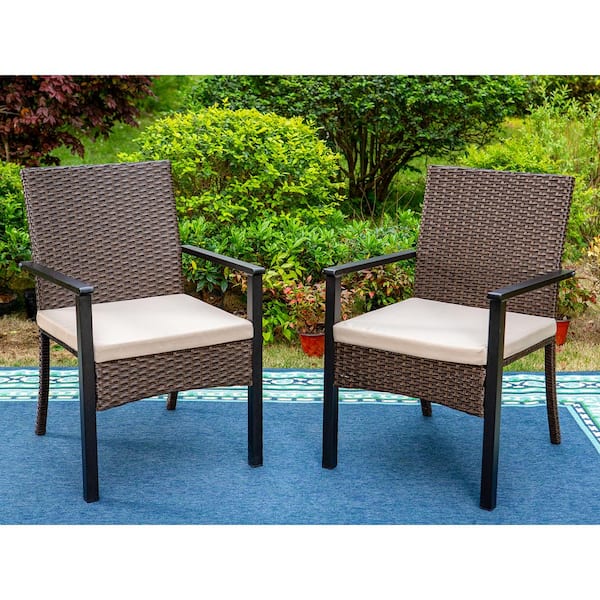This close-up product photo captures two outdoor dining chairs positioned slightly towards each other. The chairs feature brown wicker backs with dark, nearly black wooden armrests and legs, unified in a continuous design. Each chair is equipped with a square, thin white cushion on the seat, adding a touch of comfort. The lower front of the chairs shows a rectangular wicker piece connecting the legs. They rest on a blue carpet with a light blue border, placed in an outdoor setting. The background includes a lush landscaped area featuring large trees and a series of small red ceramic flower pots, each filled with vibrant, colorful plants.